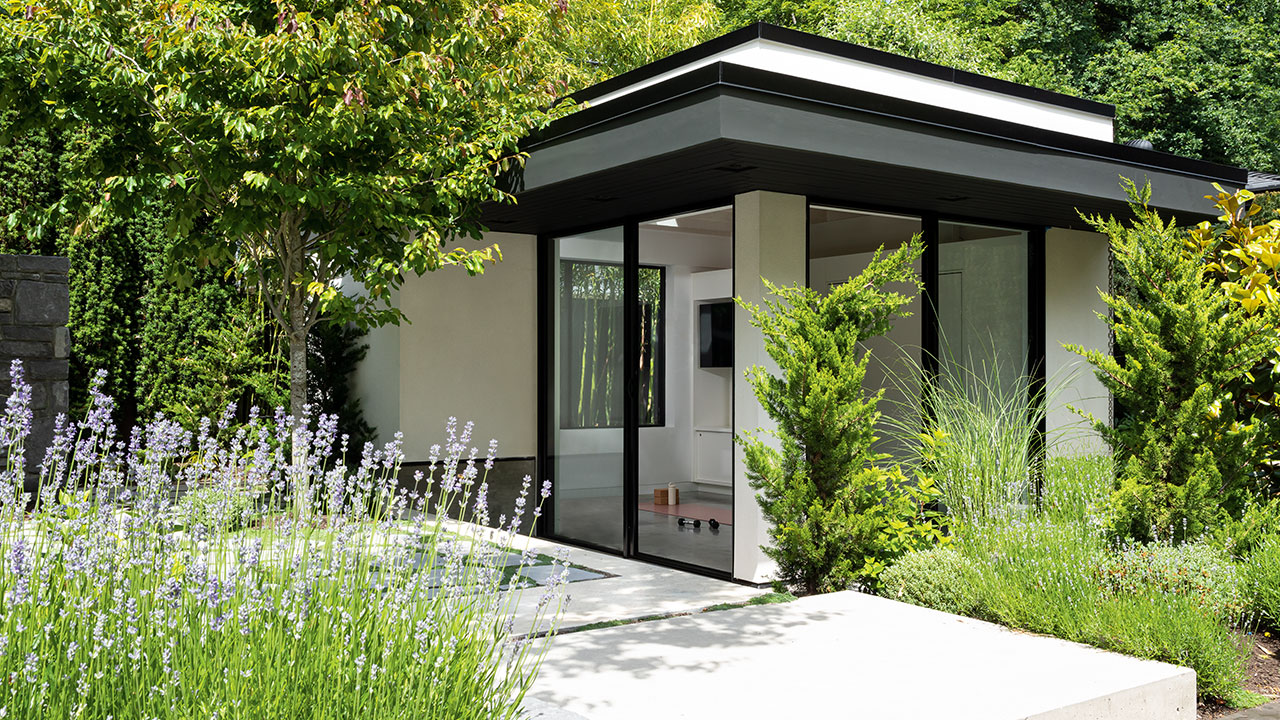In this landscape-oriented photograph, we see an ultra-modern home nestled within a lush, verdant setting. The residence features a distinctive architectural design with a flat, silver roof trimmed in black, topped by an additional flat white roof also accented in black trim, giving the appearance of two stacked roofs. The building is primarily constructed of glass, allowing a view into its interior, which includes a large framed poster with green and brown hues. The house's structure is framed with black borders and white walls that create a striking contrast to the glass.

The scene around the house is brimming with dense vegetation; towering green trees and thick, low-lying plants create a rich tapestry of greenery, interspersed with wildflowers. To the right, the vegetation consists of dense, piney trees and various plants, creating a shaded area with visible shadows. To the left, tall grass with light purple flowers punctuates the landscape. A white sidewalk and patio stones lead up to the house, accompanied by a large white patch of cement with stairs in the bottom right corner and a decorative concrete slab partially hidden by the purple flowers in the center. The house seems almost hidden among the thriving plant life, with no sky visible through the dense canopy of trees overhead.